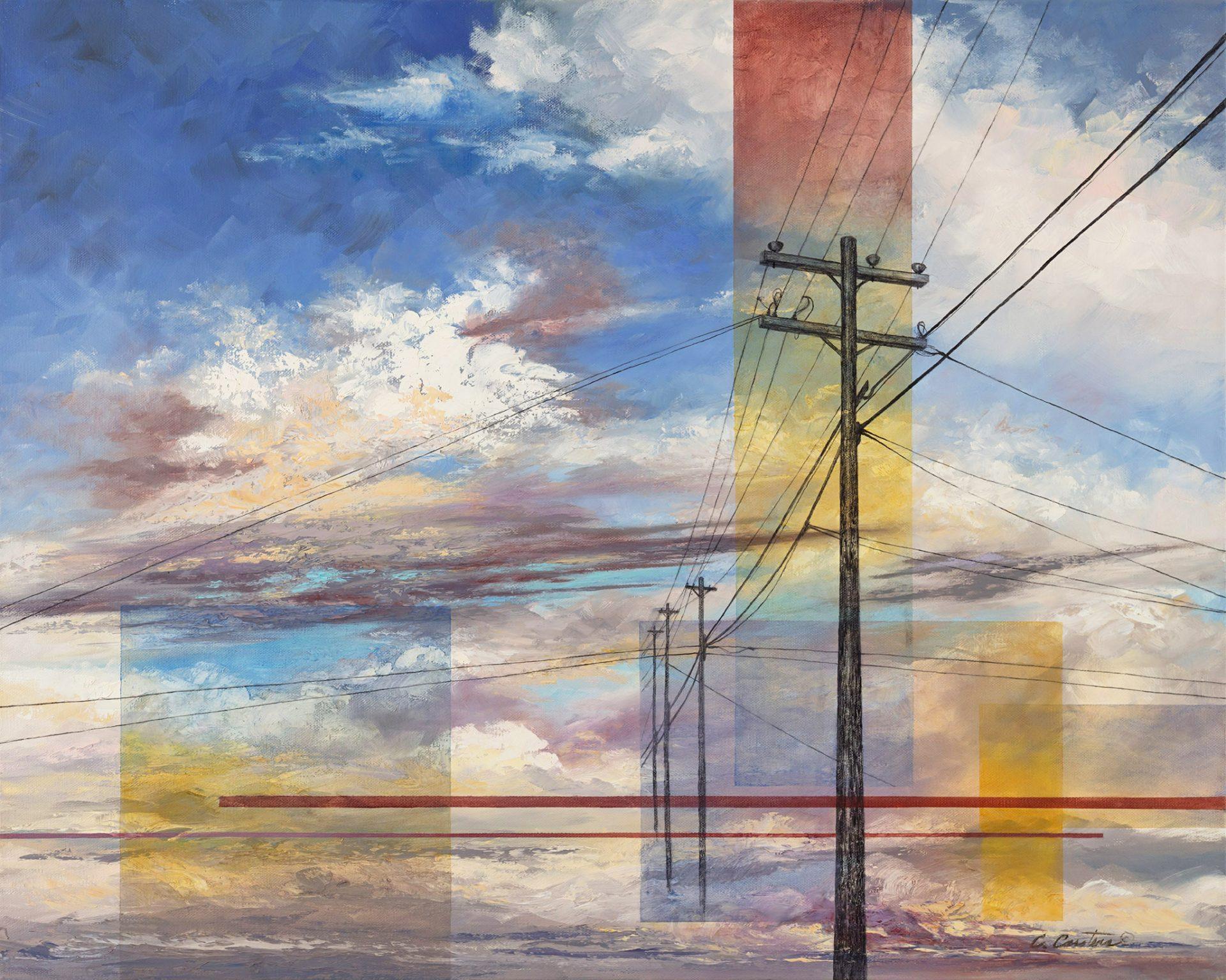This detailed painting depicts a scene dominated by telephone poles and power lines against a dramatic sky. The main telephone pole, situated slightly to the right of center, features two crossbars with insulators and extends upwards, punctuated with wires stretching in various directions, including into the distance where three more poles stand. These distant poles, each with a single crossbar, are connected by the same intricate web of wires. The sky, a significant element in the composition, is a vibrant mix of blue, white, yellow, and brown clouds, creating an ethereal backdrop. This sky is further accentuated by superimposed, translucent rainbow-colored squares that overlay the clouds, adding layers of reds, yellows, and blues that transition smoothly across the spectrum. The painting, a perfect blend of realism and abstract art, features subtle details like a faint outline of a white mountain in the lower right corner, grounding the piece in a quasi-realistic landscape. The colors and composition suggest an oil or acrylic medium, with the entire scene framed in a slightly longer-than-tall rectangular format.